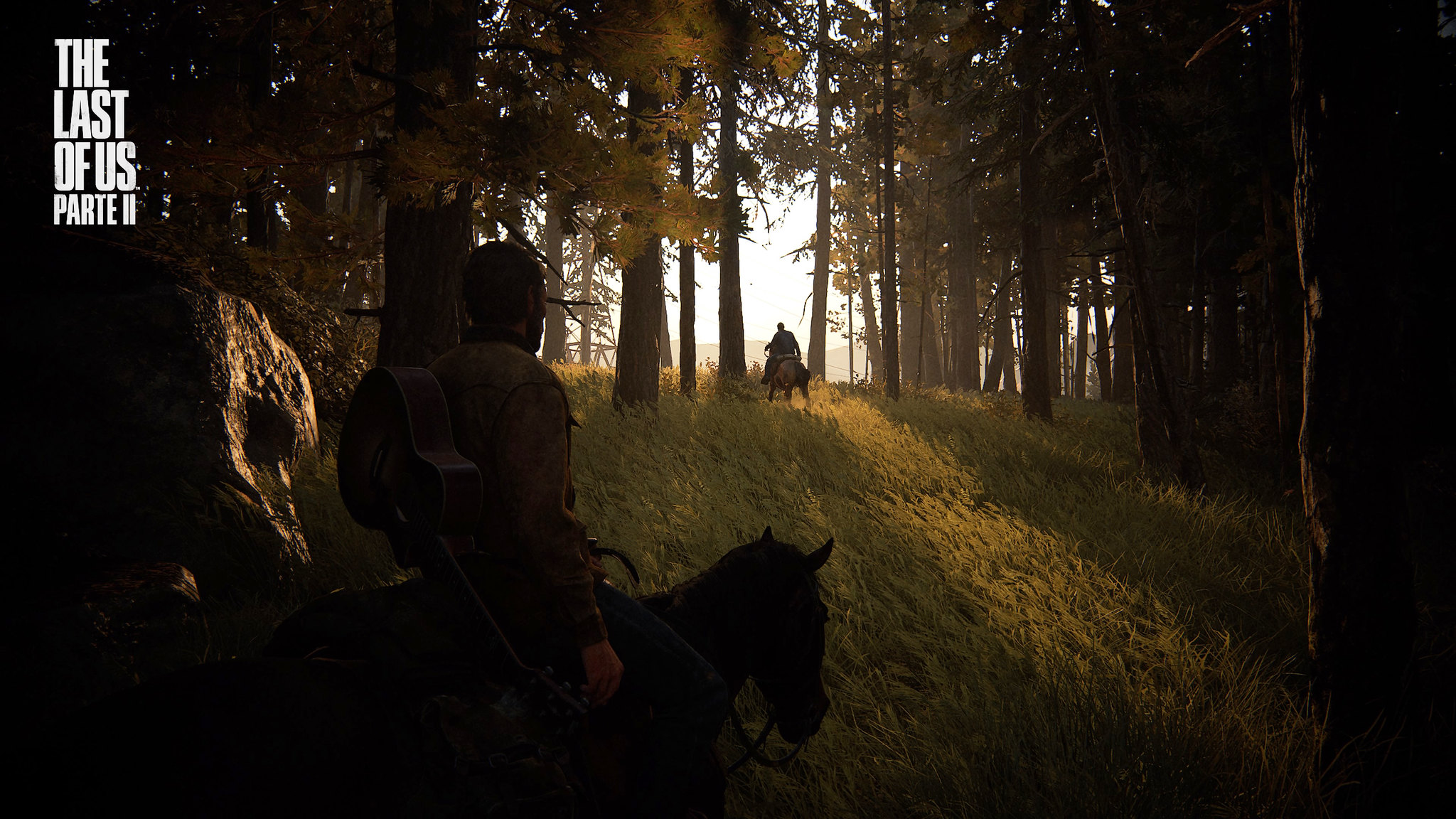This landscape image is a promotional still from The Last of Us Part 2, with the game title "The Last of Us Parte 2" displayed in the top left in Spanish. It depicts two men on horseback amidst towering pine trees, bathed in striking contrasts of light and shadow. The foreground features a silhouette of a man, likely Joel, riding a brown horse with a guitar on his back. He faces another rider deeper in the background, just emerging from the dense copse into a bright, sunlit clearing. The scene is visually dramatic, with rays of sunlight penetrating through the dark canopy, illuminating the flowy, green grass. The image captures a moment of transition as the two horsemen prepare to exit the shadowy woods and step into the light, symbolizing a journey forward.